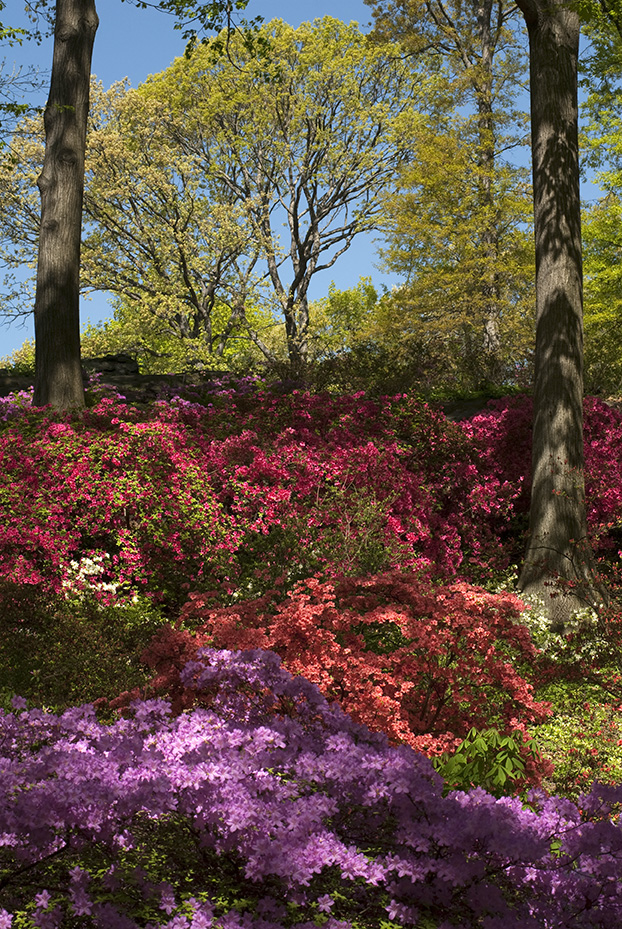This vibrant photograph, reminiscent of a magazine cover, captures a lush hillside adorned with a vivid array of flowers bathed in sunlight. Starting from the base, the hill is blanketed in a colorful progression of flowers with delicate, tiny blossoms. The foreground showcases purple or lavender flowers, transitioning to coral, then a prominent row of orange to red flowers. Higher up, the scene is dotted with bright pink flowers and lighter pink ones on the left side. Nestled among the floral display, a striking tree stands prominently on the left with another tree noticeable above it, and a third tree slightly below and to the right. The upper portion of the photograph reveals a canopy of trees with light green leaves, through which the clear blue sky is visible. Light filters through the foliage, casting intricate shadows on the ground and the trunks of the trees, enhancing the picturesque and serene atmosphere of this sunny day.